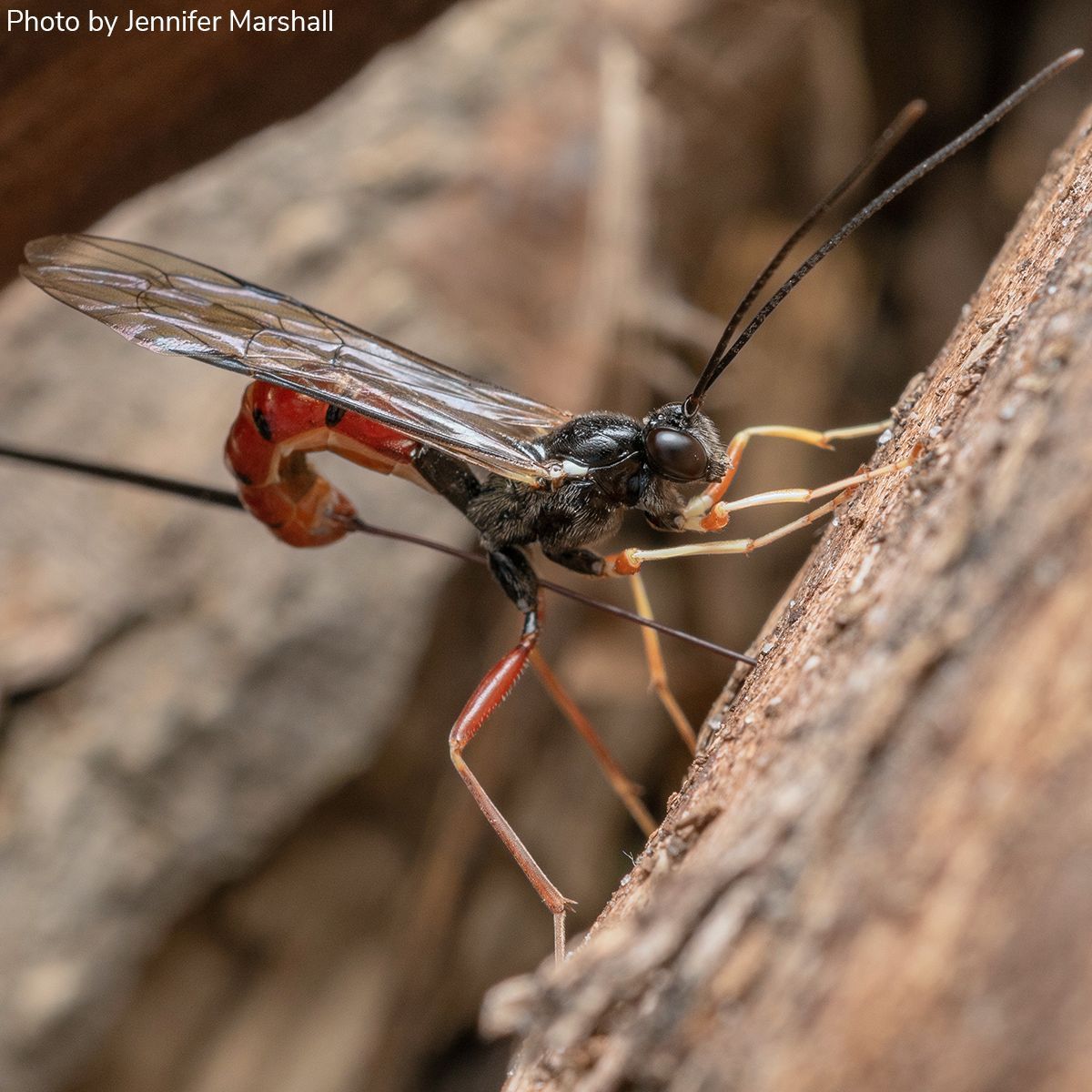The image depicts a close-up of a vibrant insect on a tree, taken by Jennifer Marshall. The insect, potentially a mosquito or a flying ant with some features resembling a bee, is centrally positioned with its face toward the bark. The insect boasts extraordinarily long black antennas and bulging brown eyes that appear larger than its tiny, round head. It has a short torso and an elongated, curled red abdomen with a long needle-like protrusion at the tip, seemingly penetrating the tree bark. Its two long, transparent wings accentuated with black jut out behind it. The insect’s legs, a mix of yellow, orange, and reddish hues, are spread at an angle as they grasp the tree bark. The surrounding environment includes tan and brownish tree bark and an out-of-focus wood bark in the background. The color palette of the photograph includes rich reddishes, black, brown, yellows, and translucent elements, enhancing the detailed and vivid portrayal of the insect in its natural habitat.